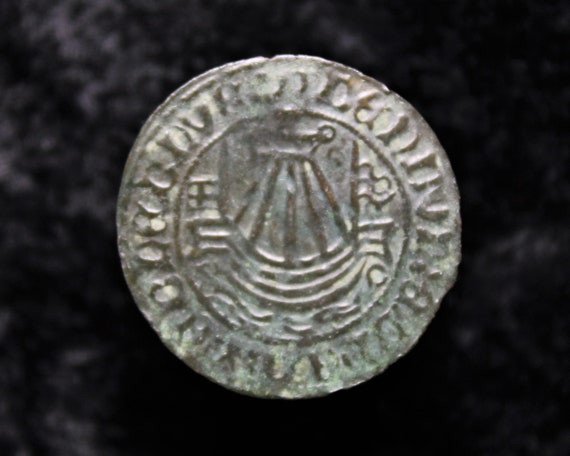This photograph features a very old, silver coin set against a black background. The coin, roughly the size and shape of a quarter, appears heavily worn and chipped around its edges, with a notable amount of rust and wear. An outer ring adorned with faded symbols, some resembling letters such as "V" and "O," encircles the coin. The text, possibly in an archaic or foreign script, is difficult to decipher, especially where it blends into areas marred by blueish discoloration.

Dominating the center of the coin is a complex design that features what appears to be an anchor shape in the upper half, accompanied by a series of five lines extending from a small box above it, lending a darker tone to the surrounding space. Below the anchor, wavy lines fill the area, escalating into more pronounced waves toward the bottom, adding to the maritime theme. Additional features include a small square window-like shape to the left of the anchor and three wavy strings to the right. The coin's intricate and ancient appearance, along with its ambiguous inscriptions and central maritime imagery, underscores its historical and enigmatic nature.